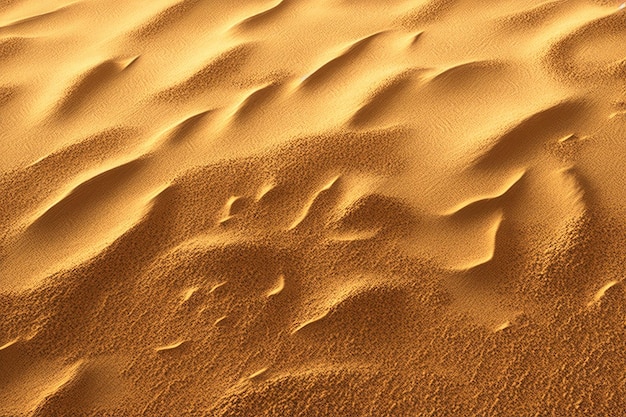This image depicts a pristine expanse of desert sand, extending seamlessly across the scene with intricate natural patterns sculpted by the wind. The sand varies in color from a rich beige camel hue to a brighter yellowish-orange, indicative of strong sunlight striking from above. The texture of the sand is notably smoother at the top left, transitioning to a rougher and more coarse appearance towards the bottom right, suggesting greater wind activity in that area. The surface is adorned with subtle wavy ridges that enhance its clean and undisturbed look, capturing the essence of an arid desert landscape under daytime illumination.